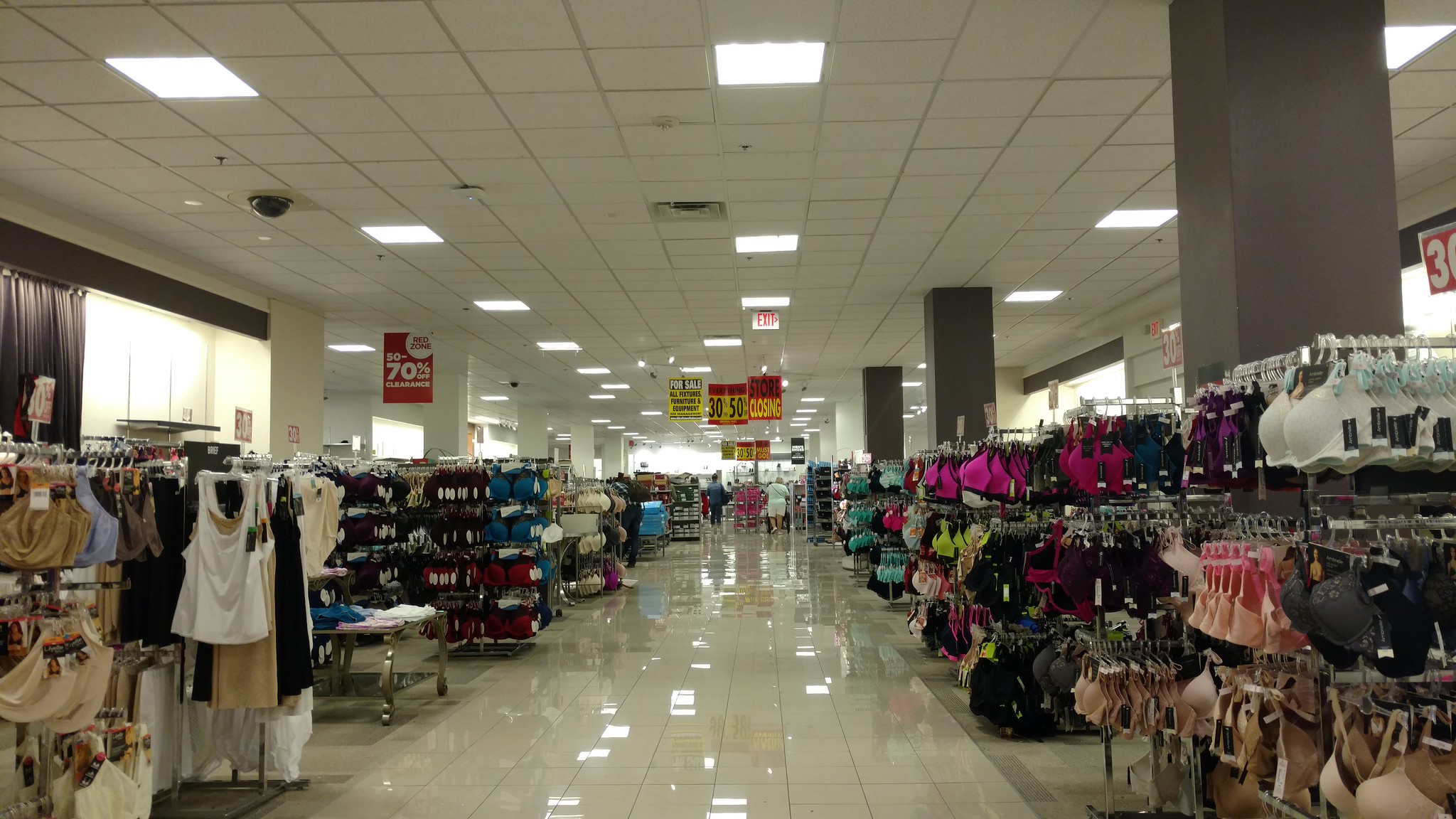A bright and glossy center aisle stretches through a department store, reflecting the overhead fluorescent lights from the white drop ceiling. The ceiling features rows of lights, evenly spaced, illuminating the scene below. Both sides of the aisle are lined with women's apparel, primarily showcasing bras, lingerie, and various tops. Interspersed among the clothing racks are tall, rectangular pillars, either dark gray or white. Near the end of the aisle, a small group of people can be seen.

Hanging from the ceiling are numerous signs, mostly in red and yellow, signaling various discounts and sales events: "30 to 50% off," a "store closing" notice, and a prominent "70% off" sign. Another yellow sign with black lettering reads "for sale," though the rest of the text is unreadable. An exit sign is visible about midway down the aisle.

Overall, the scene reflects the bustling, sales-driven environment of a department store nearing closure, with detailed focus on the sales signage and layout of the women's clothing sections.